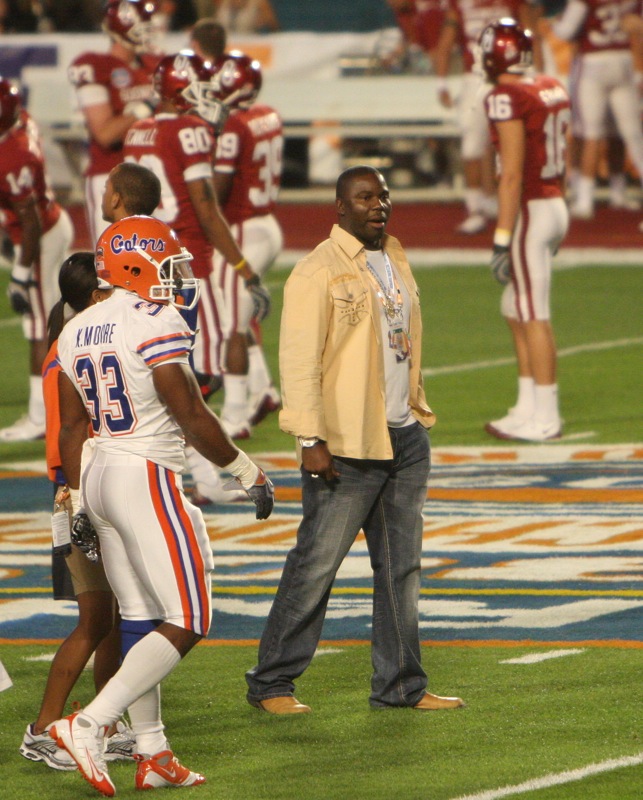This nighttime photograph captures an intense moment on a football field, illuminated by stadium lights. The focus is an African-American man, possibly a coach or official, standing prominently at a three-quarter angle facing right. He is middle-aged, sporting a light brown fade haircut, and is dressed in a white t-shirt with an indistinguishable graphic underneath a yellow long-sleeve collared shirt, dark blue stonewashed jeans, and light brown leather loafers. Around his neck, he wears several chains. 

To the left, a uniformed football player in profile catches the eye. This player is wearing an orange helmet with "Gators" inscribed on it, a white jersey accented with blue and orange, and white athletic pants. The jersey number 33 is visible, though the name on the back is too hard to read. 

In the blurred background, at least six other players in dark red jerseys with white lettering and white pants with red stripes can be seen. The field itself is marked with lines and an indistinguishable colorful logo at its center, hinting at spirited logos and team markings. Further back, the silhouettes of spectators and a stadium structure loom, accentuating the lively atmosphere of the game.